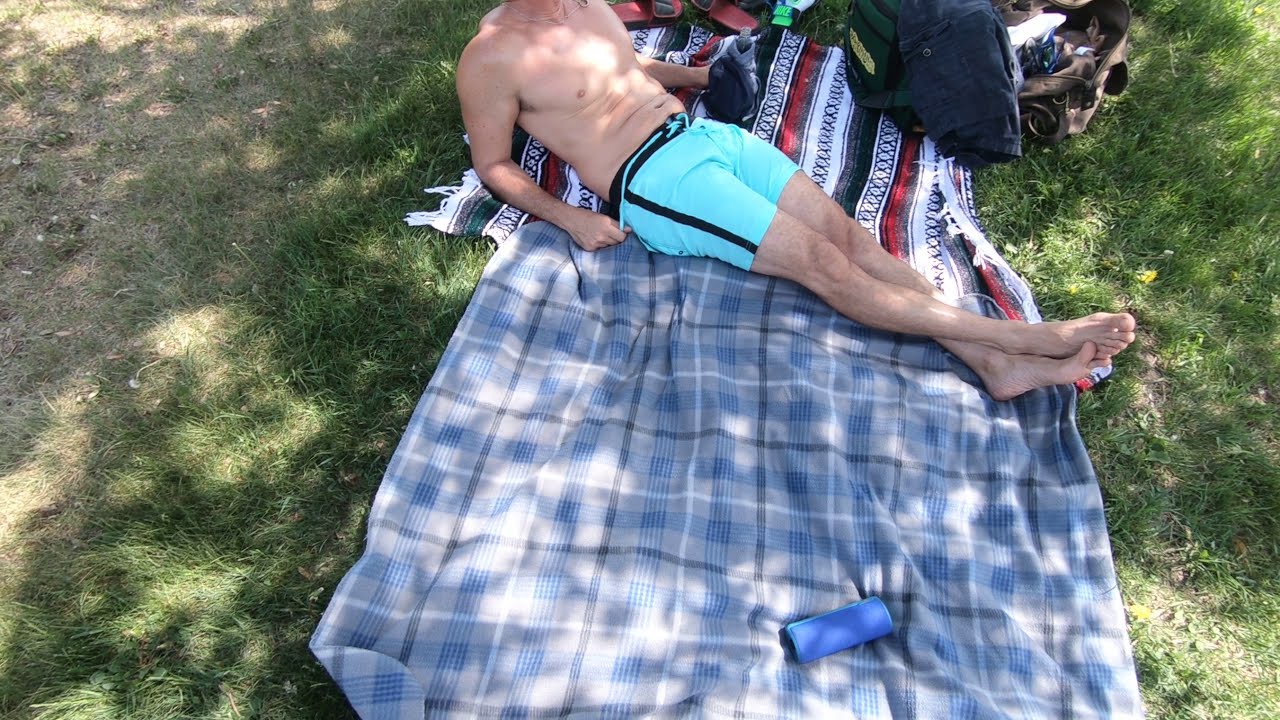The image captures a serene scene in a park, showcasing a shirtless man lounging comfortably on two blankets spread over green and brown grass. The man is dressed in light green and black swim trunks, possibly with a shade of light blue, and is bare-footed, lying on a top blanket that is white, red, black, and striped. To his right, there's a brown bag and what seems to be a silver water bottle. Below him, on a second blanket that is plaid in blue, gray, white, and black, there is a small Bluetooth speaker positioned towards the bottom of the image. The man appears relaxed, possibly enjoying a drink from a glass bottle wrapped in something, while partially shaded by a tree, indicating he is not fully sunbathing. The overall setup suggests a relaxed picnic or a leisure day spent enjoying the outdoors, enveloped in the natural colors of the park under the daytime sun.